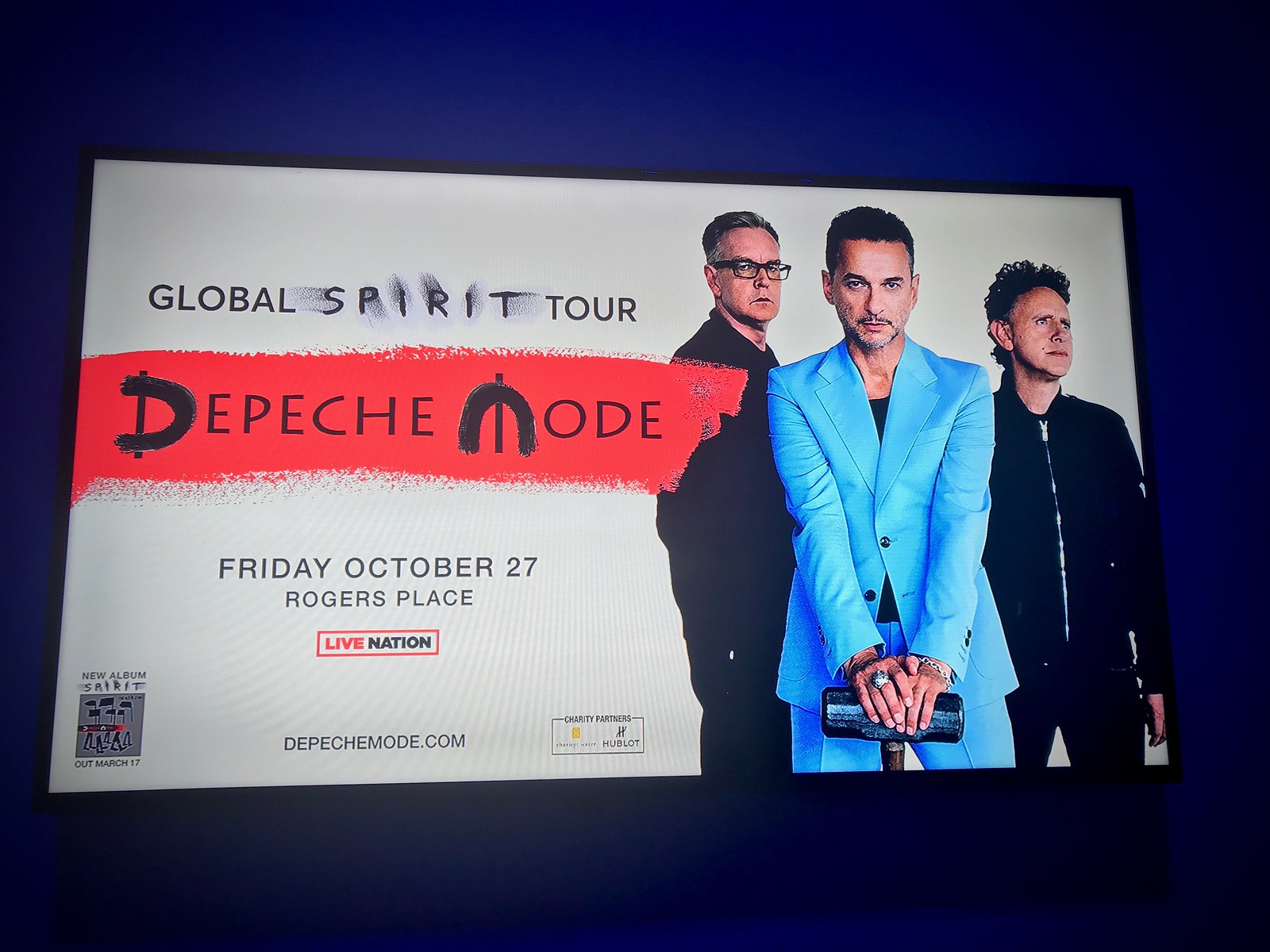The image centers on a single object framed by a very dark navy blue background. This object, likely a poster or a TV, is positioned directly in the middle of the image. The poster itself features an advertisement for the "Global Spirit Tour" by Depeche Mode, with detailed event information stating "Friday, October 27th, Rogers Place, Live Nation, DepecheMode.com," alongside logos and mentions of charity partners Hublot and Charity Water. 

The poster has a thin black frame and showcases three men on the right side: one wearing glasses and frowning, another in a black zip-up sweater with curly black hair looking away, and a third man in front, resting on a sledgehammer, adorned with rings and dressed in a light blue suit. The colors in the poster include dark blue, gray, black, red, light blue, and yellow, standing out against the dark background. This advertisement promotes the tour and the band's new album, "Spirit," released on March 17.